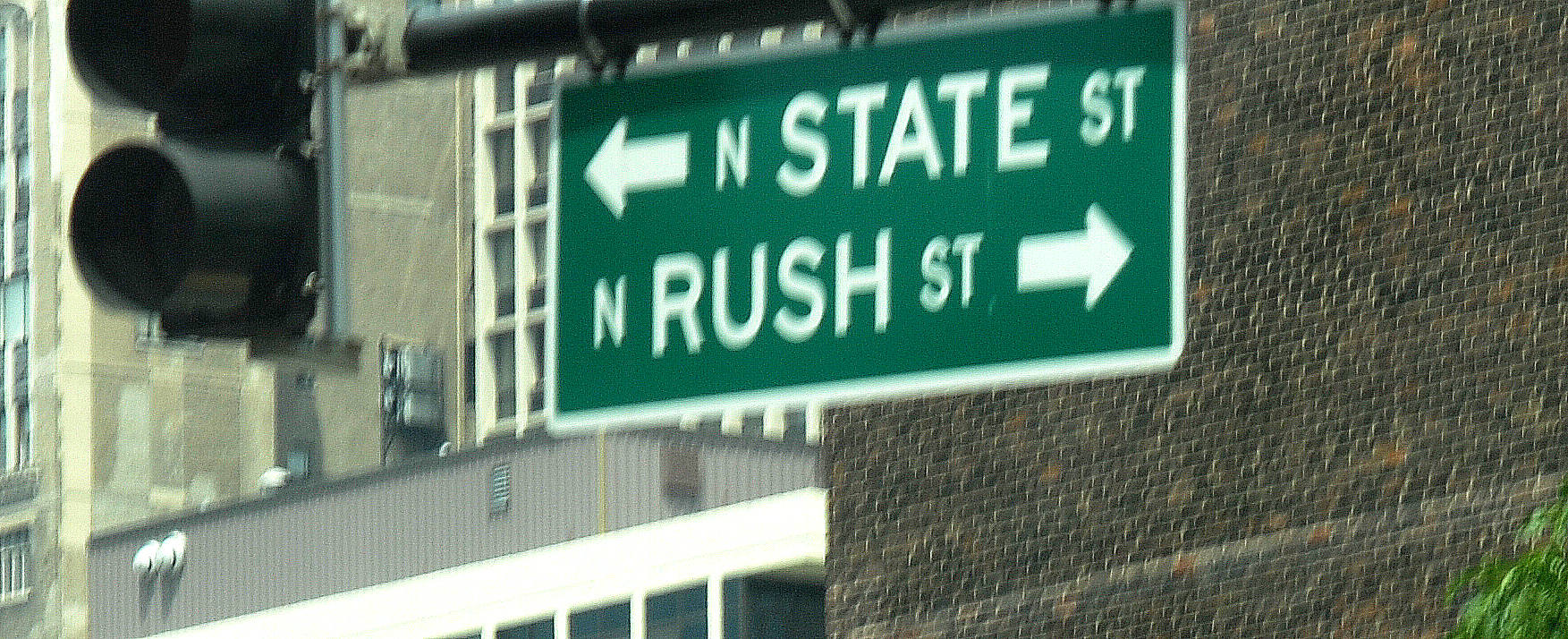This long and narrow photograph, taken in landscape orientation, captures an urban scene through an upward, exterior perspective. The image is somewhat blurry, suggesting motion or a low-quality capture. In the distance, two large buildings dominate the view: one is constructed from brown brick, while the other is a light-colored stone edifice with numerous windows. Prominently featured in the foreground is a black traffic light, from which a green road sign with white lettering is suspended. The sign indicates "N State Street" and "N Rush Street," with arrows pointing in different directions to guide traffic. The photograph appears to be a cropped segment of a larger original image, adding an intriguing sense of context and depth to the urban landscape.